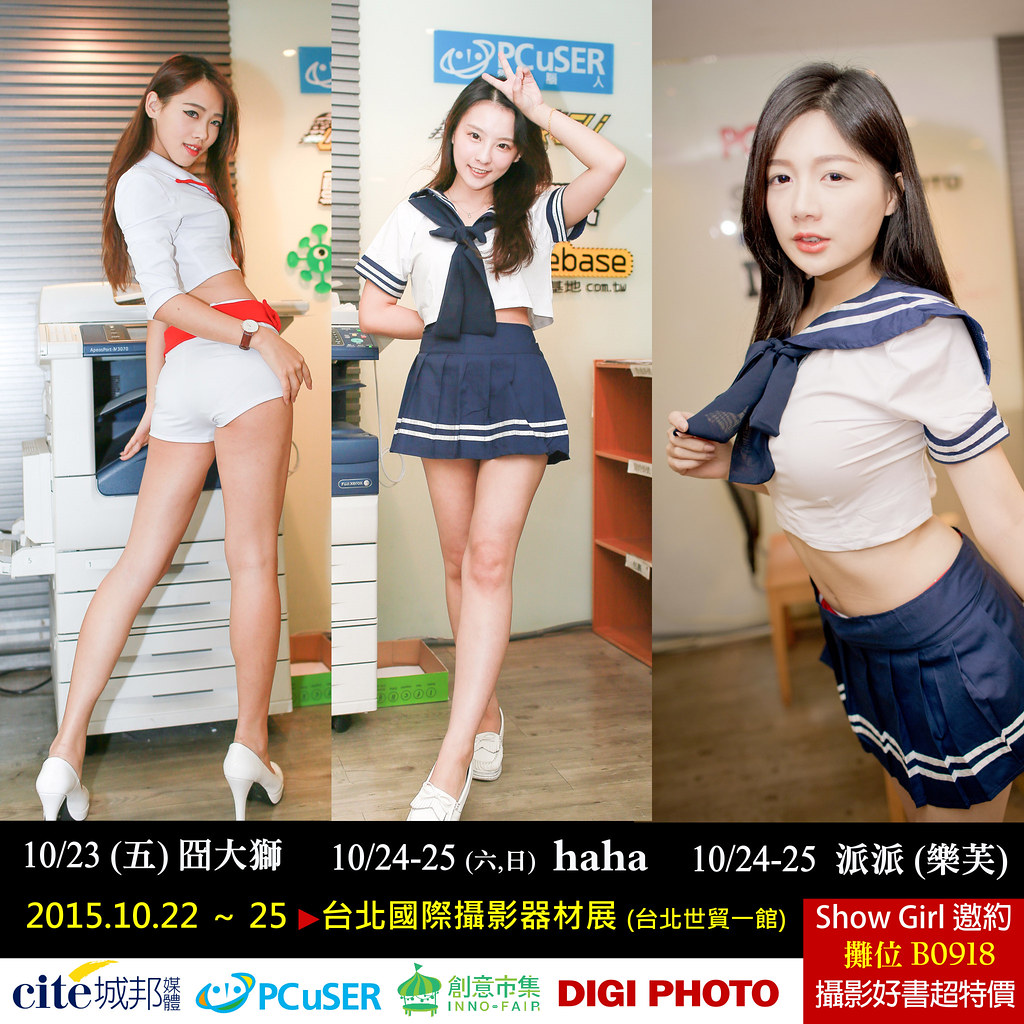The image appears to be an advertisement, likely from an East Asian context, featuring a collage of three photographs of young women dressed in provocative outfits. Each photograph showcases an Asian woman with long hair, and they are all positioned inside an office-like environment. 

From left to right:
1. The first woman, standing front of a copier, is turned towards the camera. She has long brown hair and is dressed in a white crop top and short white shorts with red trimming at the top, complemented by white high heels.
2. The second woman, centrally located, has long brown hair and strikes a pose with her left arm raised, forming a peace sign on her forehead. She dons a sailor-style ensemble consisting of a white and navy blue top paired with a short blue skirt edged in white, and she also wears white shoes.
3. The third woman on the right has long black hair and looks straight at the camera, wearing a similar navy sailor outfit with a short blue skirt and a white top highlighted by a blue accessory around her neck.

Text in Asian characters, interspersed with dates indicating "1023," is displayed beneath the images. The bottom right corner of the advertisement contains a red box with the word "Showgirl" written inside it, likely in Chinese characters, accompanied by additional yellow and white text below. Various logos and brand names are scattered along the lower left part of the image, adding to the promotional feel of the advertisement.